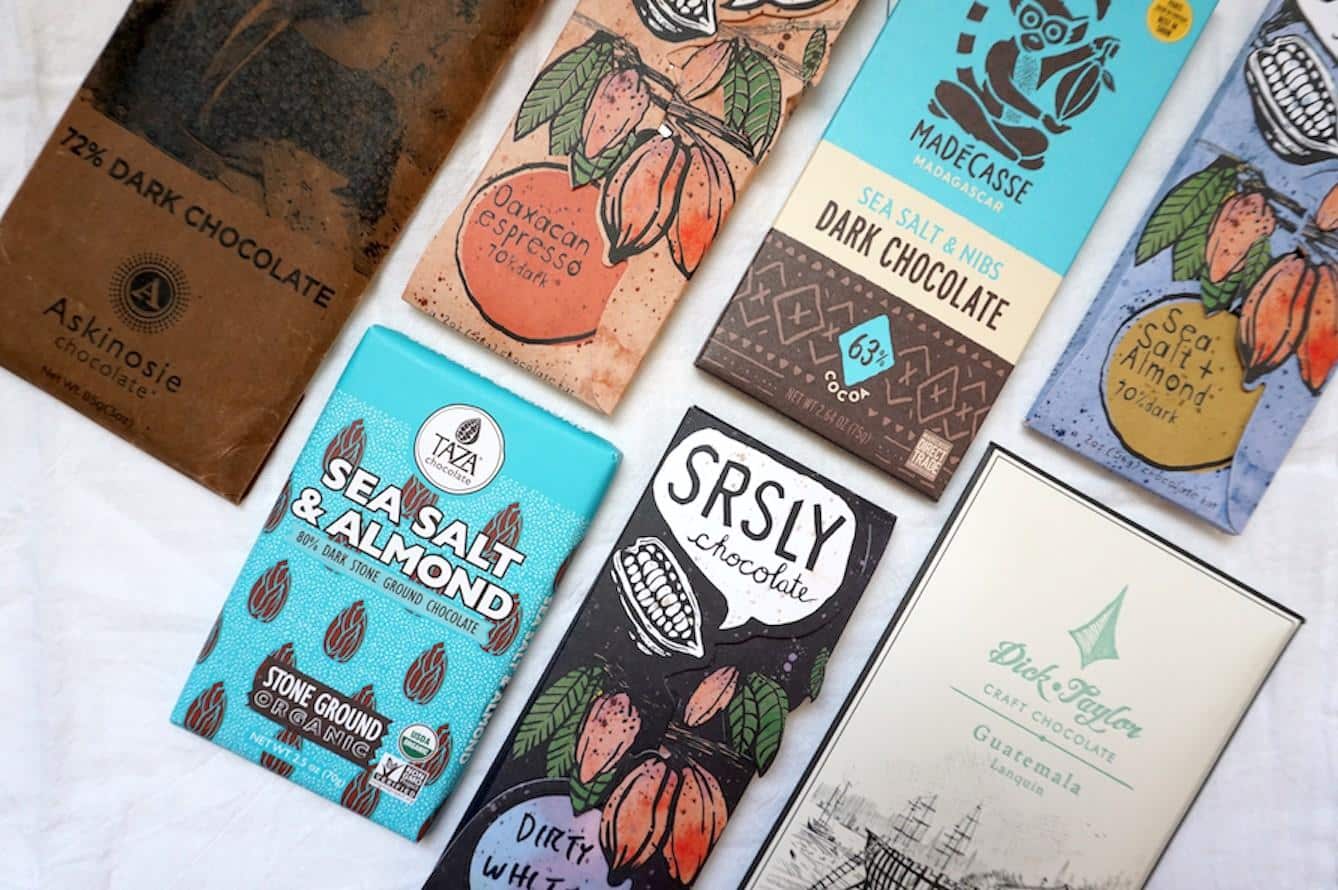This is a detailed color photograph taken from a top-down perspective, showcasing an array of seven fancy chocolate bars meticulously arranged against a pale gray background. The image features two neat rows, with four bars on the top and three on the bottom, all staggered slightly from left to right. Each chocolate bar boasts its own unique, colorful wrapping, many adorned with intricate woodcut designs and artistic elements. 

Dominating the scene are various brands and flavors, including Dick Taylor craft chocolate from Guatemala, featuring bold designs. Among the selection, there's SRSLY (S-R-S-L-Y) chocolate offering a combination of sea salt and almond, and Taza's 80% dark, stone-ground organic chocolate. Askinosie’s 72% dark chocolate and their distinctive Oaxacan Espresso flavor are also highlighted, along with Madécasse dark chocolate from Madagascar, which is infused with sea salt and nibs.

The assorted packagings display clear text and labeling, listing cocoa percentages and flavor combinations such as sea salt plus almond, 63% cocoa, and 70% chocolate. The photograph is taken in bright, ample lighting, allowing each chocolate bar's intricate design and vibrant color to be captured in sharp detail, making the overall image visually appealing and easy to examine.